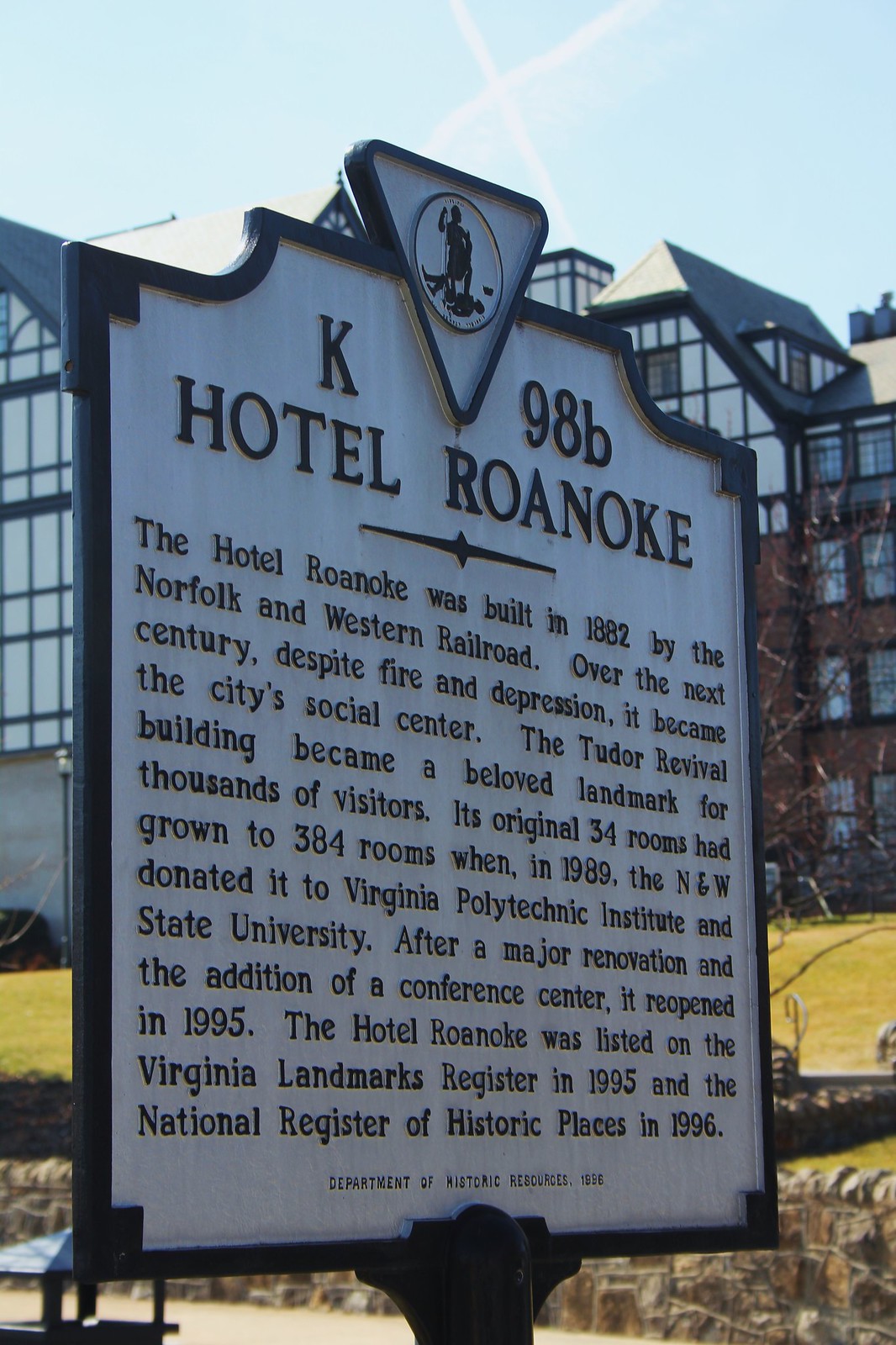This image showcases a tall, rectangular photograph of a white sign with a black metal border, prominently displayed outside. The scene captures a green, grassy sloped lawn in the background, bordered at the bottom by a gray stone wall. Beyond the lawn, multi-story buildings in brown and white with multi-layered black plaid patterns can be seen. The sign itself, tilted so that the left side is closer to the viewer than the right, dominates most of the image. It features an elaborately designed top with an inverted triangle containing a circle and a figure. 

The text on the sign reads: "K98B Hotel Roanoke. The Hotel Roanoke was built in 1882 by the Norfolk and Western Railroad. Over the next century, despite fire and depression, it became the city's social center. The Tudor Revival building became a beloved landmark for thousands of visitors. Its original 34 rooms had grown to 384 rooms when, in 1989, the Norfolk and Western Railroad donated it to Virginia Polytechnic Institute and State University. After major renovations and the addition of a conference center, it reopened in 1995. The Hotel Roanoke was listed on the Virginia Landmarks Register in 1995 and the National Register of Historic Places in 1996."

The comprehensive detail along with the historical significance of the landmark, signifies its importance and highlights its transformation and resilience over more than a century.